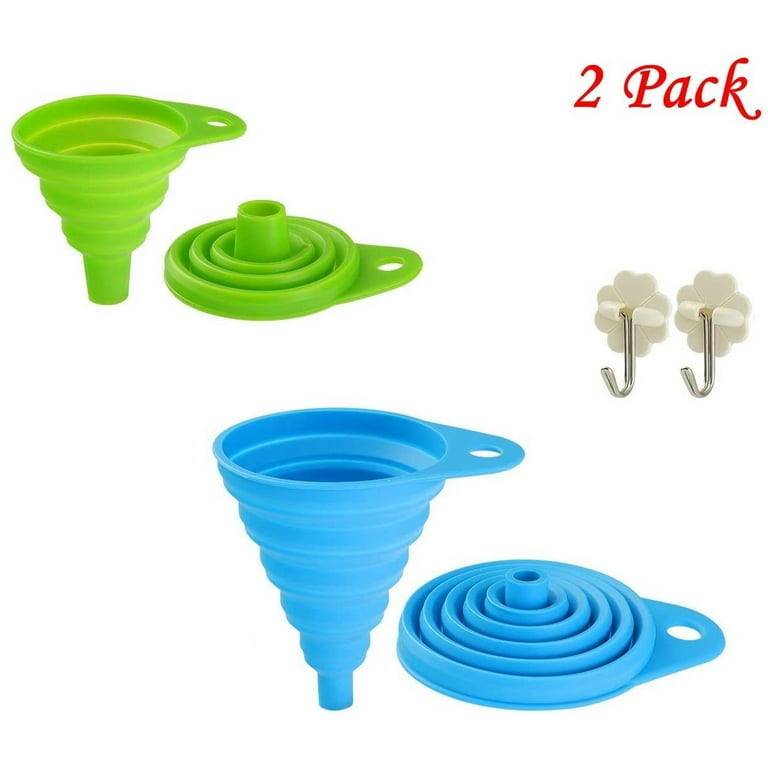This is a detailed product photo of a 2-pack of collapsible silicone funnels, advertised in red text at the front right of the image. These funnels are designed for pouring liquids into containers, suitable for tasks such as adding oil to an oil tank or transferring other fluids like steering fluid. The image showcases two funnels: a smaller green one and a larger blue one. Both funnels are depicted in both their fully spread out and collapsed forms, illustrating their versatility and space-saving design. Each funnel features a small hole on the rim, allowing them to be hung on hooks, which are also included in the product. These hooks are shown to the right of the funnels, white in color with a flower shape and a metal hanging part. The vibrant, day-glo colors of the funnels not only enhance their visual appeal but also suggest their silicone composition, ensuring heat resistance.